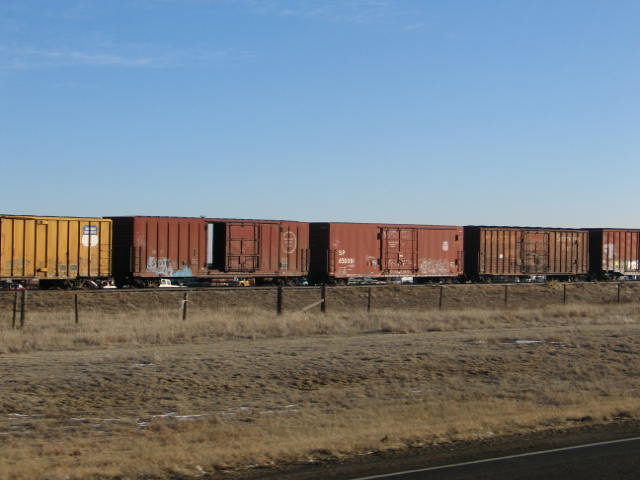This detailed color photograph captures a stationary freight train composed of five cars on tracks in a rural setting. The foreground features unkempt, beige-brown grass indicative of the season, merging into patches of green and enclosed by a wire fence. Each train car exhibits different, weathered colors starting with a yellow car on the far left, followed by a dark brown car with an open door. Next are two more dark brown cars with closed doors, with the final car, partially visible, being a red hue. The train cars appear aged but relatively free of graffiti, except for a small blue spray-painted section on the second car from the left. In the background, a vast, clear blue sky transitions to almost white at the horizon, suggesting the photo was taken in the morning with sunlight illuminating the scene from the right. A small portion of dark asphalt highway is visible in the lower right corner, adding to the composition’s depth. The photograph is devoid of human presence, emphasizing the solitary and rustic nature of the environment.